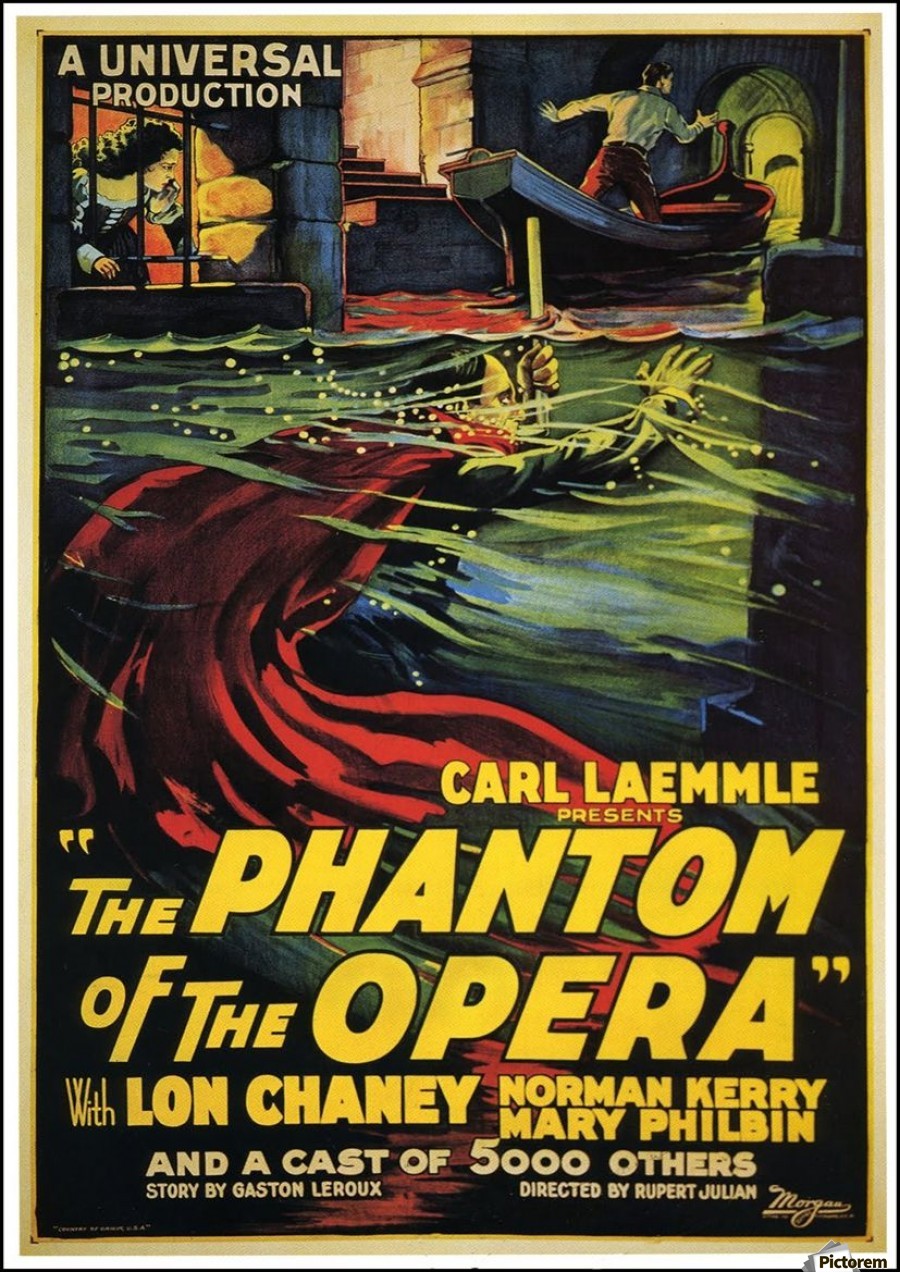This vertically-oriented, vintage movie poster is framed by a black line defining the outer rectangle, followed by a white border and a golden or beige border. Within the golden border at the top, in a beige or golden hue, it reads, “A Universal Production." Dominating the poster is a colorful illustration from "The Phantom of the Opera." The striking artwork depicts a man, presumably the Phantom, emerging from water, his long red cape billowing fluidly around him and accented with swirling white circles. In the backdrop, a woman with long dark hair peers out from behind a barred window, while a man stands on a boat that appears to be approaching a tunnel or staircase, with the water around it tinged red.

At the bottom of the poster, bold yellow text announces, "Carl Laemmle presents The Phantom of the Opera," followed by the names "Lon Chaney, Norman Carey, and Mary Philbin." Beneath this, in a lighter cream color, it states, "and a cast of 5,000 others," along with "Story by Gaston Leroux, directed by Rupert Julian." A signature, seemingly reading "Morgan," is visible towards the bottom right above the outer black frame, which also features the word "pictorum."